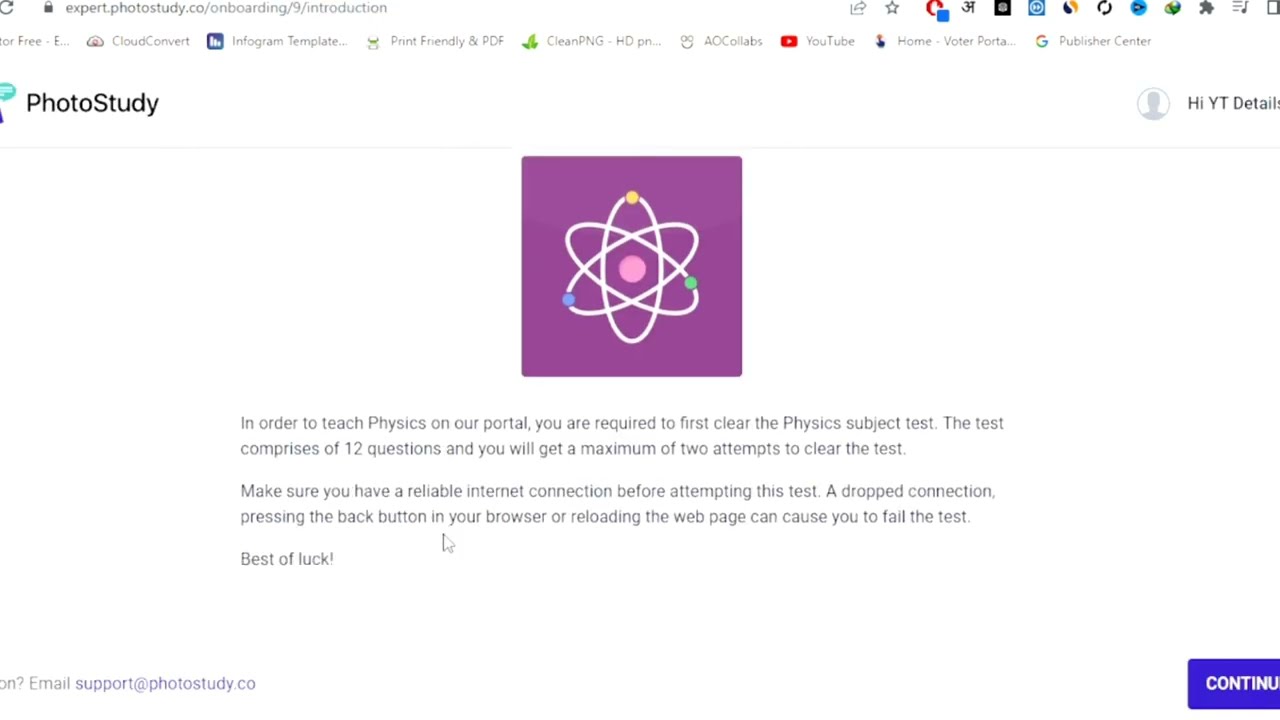This is a detailed screenshot of a web page from a Chrome browser. At the top, we see the address bar displaying the URL "expert.photostudy.co," flanked by several extension icons to the right. Below the address bar is the bookmark bar, populated with various bookmarks. The main content area starts below, featuring a white background.

On the top left of the web page, the title "Photo Study" is visible. Centrally positioned is an image of a nucleus or atom, detailed with colored dots—yellow, green, blue, and a pink dot in the center—enclosed within a purple square. Below this image appears a text section in black font, which reads:

"In order to teach physics on our portal, you are required to first clear the physics subject test. The test comprises 12 questions, and you will get a maximum of two attempts to clear the test. Make sure you have a reliable internet connection before attempting this test. A dropped connection, pressing the back button in your browser, or reloading the web page can cause you to fail the test. Best of luck."

An email support contact "support at photostudy.com" is mentioned on the left, and at the bottom right there's a blue "Continue" button, indicating a prompt to proceed. Overall, the screenshot captures a training or onboarding interface on a user's computer screen.